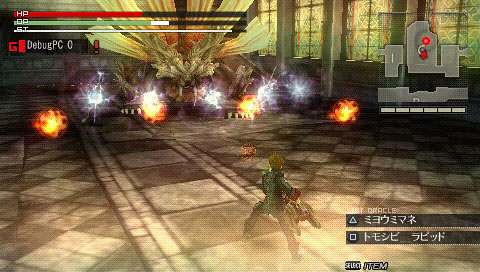This still frame from a video game captures an intense moment of action. Dominating the foreground is a patterned brown argyle floor, a unique blend between an argyle and checkered design. At the center of the frame, we see a character—likely the player—armed with a large gun and positioned with their back to the viewer. The character is currently aiming at a formidable enemy creature occupying a substantial portion of the upper half of the frame, which appears to be taking fire.

The photo is presented in landscape mode. In the upper left corner, various elements of the game's HUD are visible, including a red line labeled as "HP" indicating health, a green line labeled "OP," and a white line labeled "ST," likely representing different status bars. Below these is the text "DEBUG PC," which seems to be an overlay not typically part of the game's standard display.

Additional information includes Japanese characters on the lower right side of the screen, accompanied by the words "SELECT ITEM." On the upper right, a top-down mini-map provides a view of the character's location on the playing field, adding a strategic layer to the scene being viewed. The intricate details and overlays contribute to an immersive gaming experience, capturing the player's battle against a monstrous enemy in a meticulously designed environment.